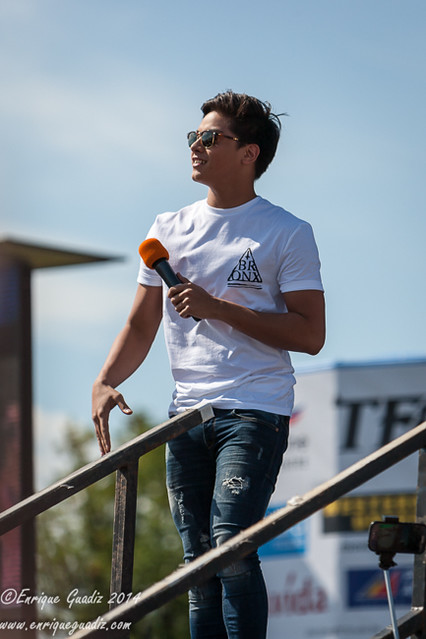An outdoor scene captures a man with darker skin and dark hair, standing near a staircase and seemingly engaging with a crowd, though the audience is not visible. The sky is a clear blue with a slight shading of blurry clouds. Background elements include signage with partially readable text "TE" and various logos, including a TF and a Western Union icon, with trees and possibly a building partially out of focus. The man, framed at the forefront, is smiling and looking slightly upwards to the left. He wears brown sunglasses, a white short-sleeve t-shirt with a triangular graphic and the word "Bronx" on it, and ripped jeans. Holding a microphone with an orange top, his image includes a text watermark in white indicating "copyright Enrique Enrique Gad Gad 2014" and a website "www.enriquegadis.com."